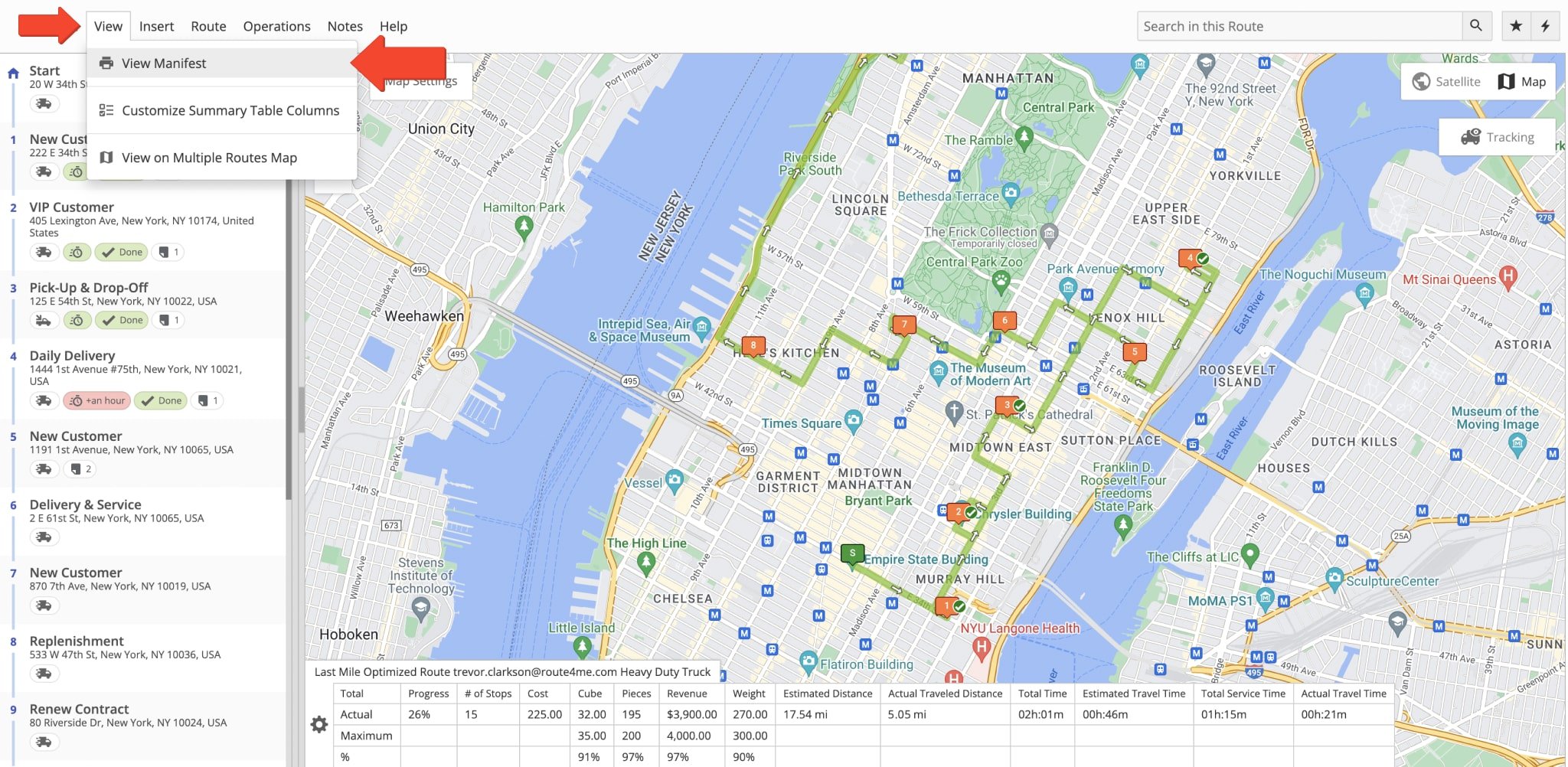The image features a detailed map with various interface elements overlaid. At the top right, there are two rectangular boxes with a gray background. The first box contains a light gray text that reads, "Search in this route," along with an icon of a magnifying glass. The second box displays a gray star, followed by a vertical line. Extending from this line is an icon resembling a lightning bolt or a backward 'Z'.

The map itself depicts a region with bodies of water on both the left and right sides. One of these bodies of water is labeled "New York, New Jersey," while the other is identified as the area around "Roosevelt Island, East River." The map also shows various streets and numerous "M" symbols, suggesting metro or subway stations, as well as bus routes.

At the bottom left corner of the map, black text reads: "Blast map, optimize route, trevor.croftson@route4me.com, heavy duty truck." On the left side of the image, there are two red arrows. One arrow points to the top tabs labeled "View, Insert, Route, Operation, Notes, Help." When the "View" tab is clicked, a dropdown menu appears, with the first option being "View Manifest," which the other arrow on the right-hand side points to. Below that, the options "Customize Summary Table Columns" and "View on Multiple Routes Map" are listed.